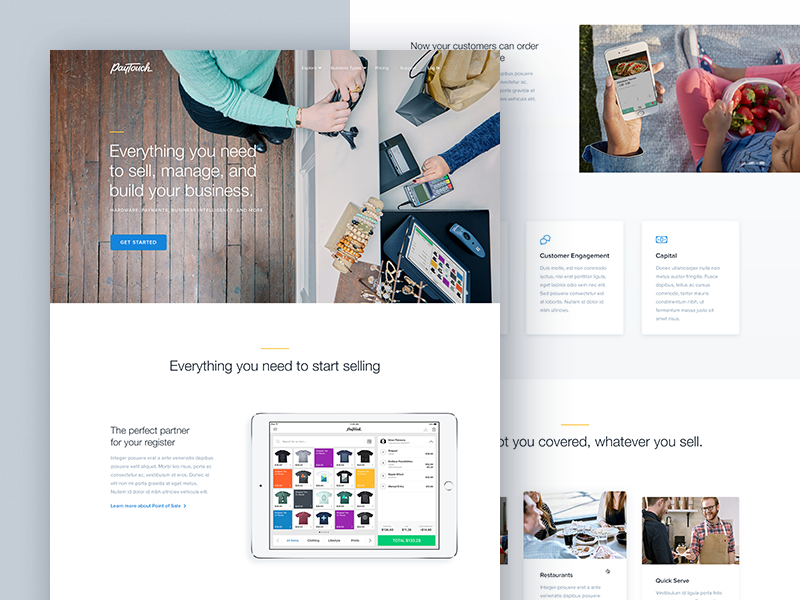Overhead shot of a point of sale (POS) system in action: A person processes a payment using a credit card, illustrating the ease and efficiency of the PayTouch POS system. To the right, a parent sits with a child on their lap, both engaged with a mobile phone, perhaps using an app connected to PayTouch. Nearby, a small Tupperware container filled with fresh strawberries adds a touch of everyday life. Key features and promotional messages frame the image, promoting the versatility and comprehensive nature of the system: "Everything you need to sell, manage, and build your business," "Perfect partner for your register," and "You covered whatever you sell." The scene underscores PayTouch as the ultimate business solution for seamless transactions and customer engagement.